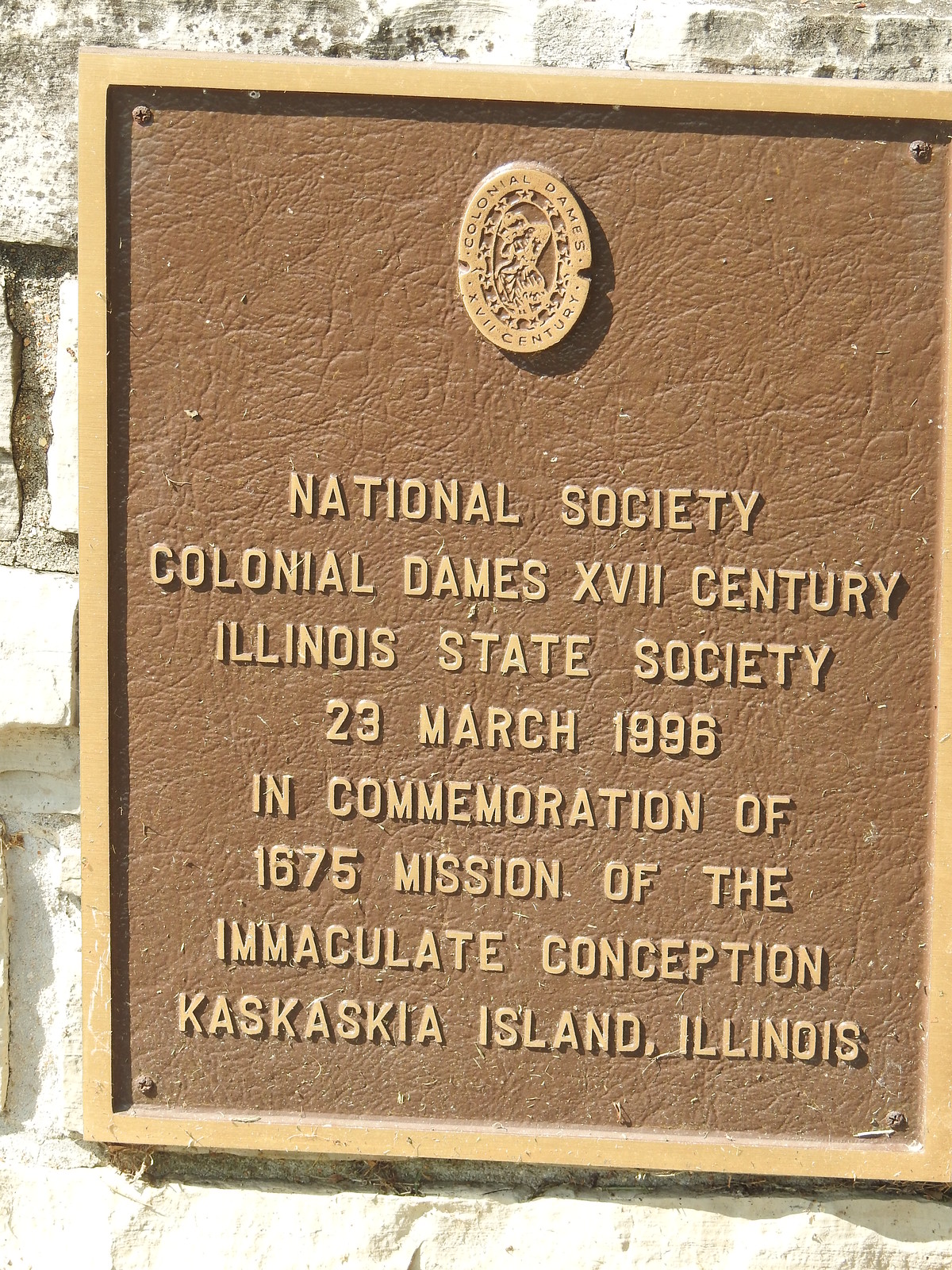The image is a close-up photograph of a commemorative plaque mounted on a light, possibly gray or chalky white, wall, which appears slightly worn and may consist of white bricks. The plaque itself is a dark brown with a light brown frame. The top third of the plaque features an oval seal, which is difficult to make out, but seems to bear the inscription "Colonel Dames" along with a date. Below the seal, in light brown letters against the dark brown background, is detailed text that reads: "National Society, Colonial Dames, XVII Century, Illinois State Society, 23 March 1996, in commemoration of the 1675 mission of the Immaculate Conception, Kaskaskia Island, Illinois." The plaque dominates the image, making it hard to discern much about its surroundings.